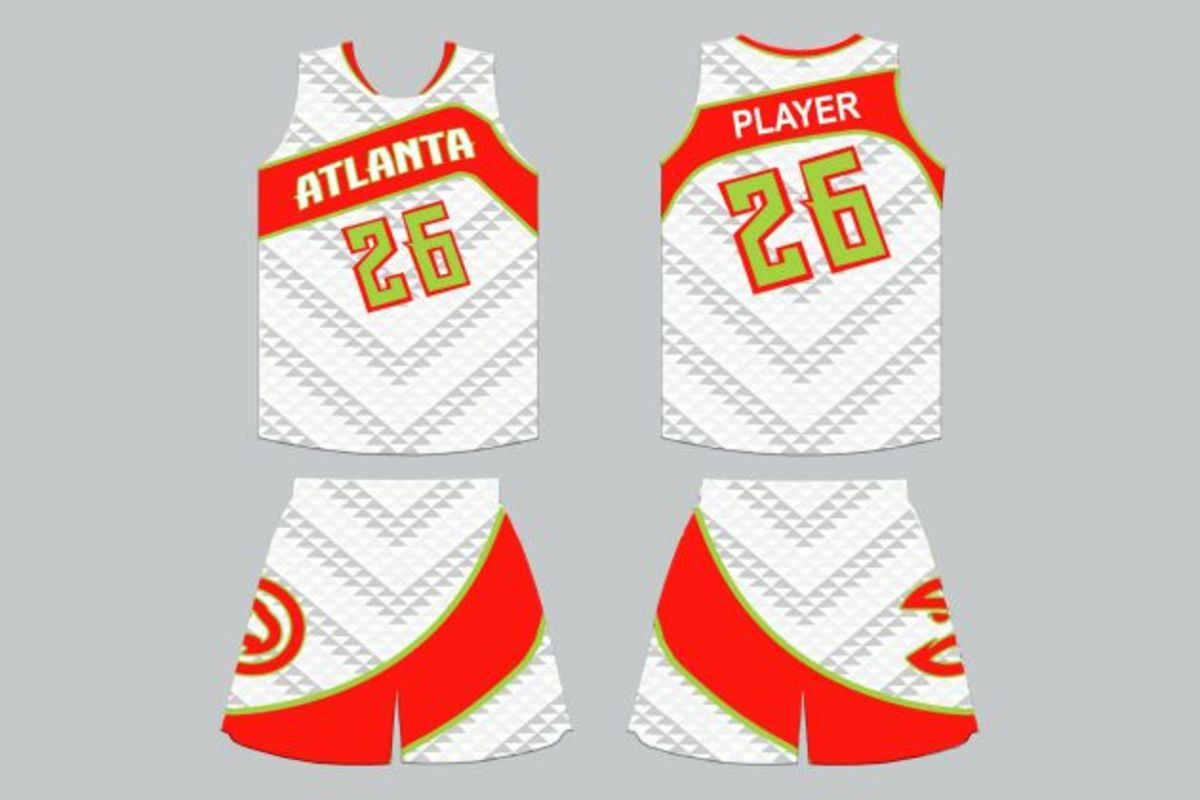This image is an illustration showcasing the front and back designs of a basketball uniform. The uniform consists of a vest-style top and shorts, both predominantly white with grey triangular details in a chevron pattern. The neckline of the top features a red border. Across the chest, there is a red banner with the word "Atlanta" in white text. Below this banner, the number 26 appears in green outlined with red. This red banner continues onto the back of the top, where it is positioned just below the shoulder blades and displays the player’s name above the green number 26 outlined in red.

The shorts complement the top with their white base and grey designs. A red swoosh extends from the bottom of one pant leg up towards the hip, revealing the edge of a circular logo peeking out. The back of the shorts shows the continuation of this red swoosh in the opposite direction and the other part of the logo on the opposite side. The uniform's cohesive design emphasizes the combination of white, grey, red, and green, integrating these elements throughout both the top and shorts for a unified look.